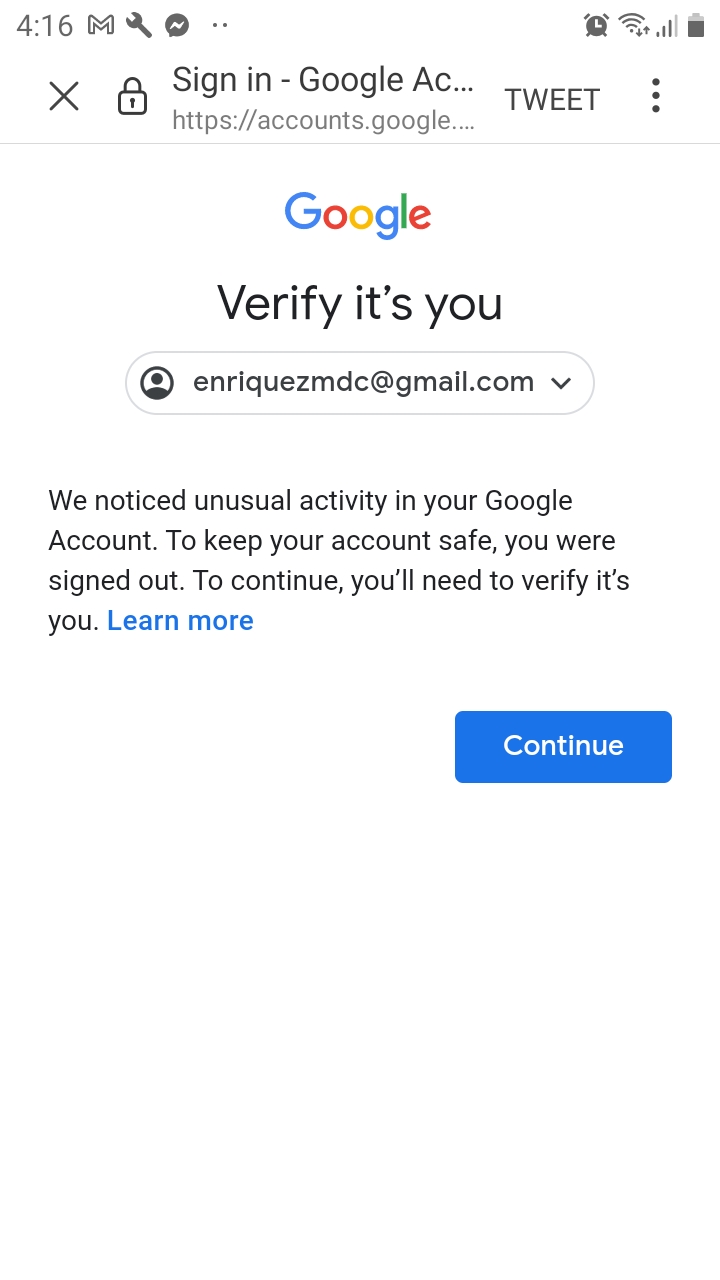The screenshot displays a cell phone screen with a predominant white background, primarily featuring text pertaining to a Google account. In the top left corner, there is the number "416", followed by a stylized "M", an image of a wrench, and a speech bubble icon. The top right corner includes an alarm clock icon, cellular connection strength bars, a wireless signal icon, and a mostly full battery indicator.

On the left side beneath this row, an “X” icon is visible next to a padlock icon, followed by the text "Sign in Google ac..." The middle of the screen prominently displays the beginning of a Google account's email address. To the right of this, there is the word "TWEET" in all capital letters.

Further down, there is a horizontal line separating the top section from the main content. Below the line, the Google logo is visible. Underneath the logo, the largest text on the page reads "Verify it's you". This section is enclosed within a bordered box.

Inside the bordered box, there is a circle containing a generic user icon, next to which the email address "enriquezmdc@gmail.com" is displayed alongside a small downward-pointing arrow. The bordered box includes the message: "We noticed unusual activity in your Google account. To keep your account safe, you were signed out. To continue, you'll need to verify it's you." Below this message, blue text stating "Learn more" is evident. On the right side at the bottom of this section, a "CONTINUE" button is present.